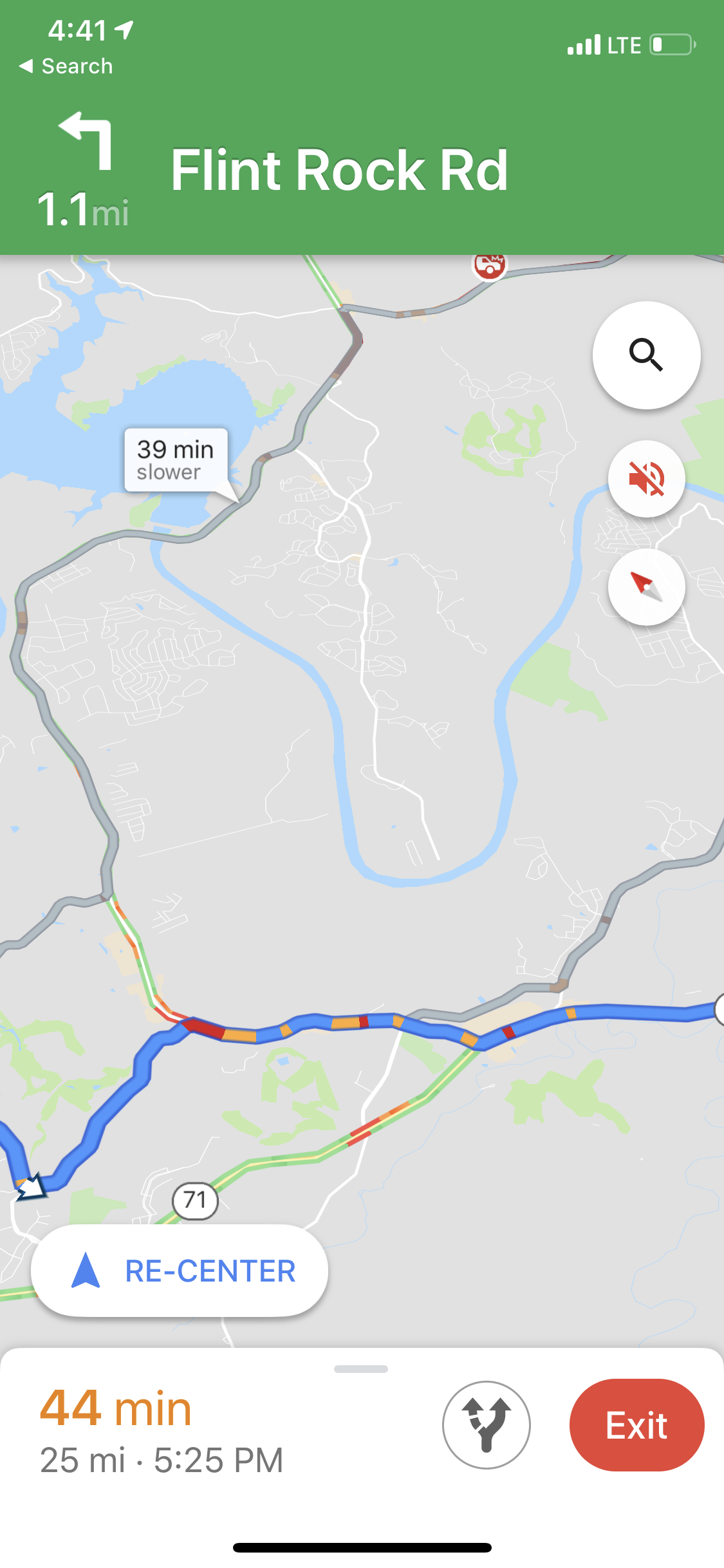The image is a detailed screenshot of a smartphone displaying a Google Maps navigation route. The top of the screen is green with white text, resembling a highway sign, and shows the user has a full LTE signal but a low battery around 20% at 4:41 PM. An arrow points northeast, indicating the direction, and the screen indicates the next turn is in 1.1 miles onto Flint Rock Road. The GPS map prominently features roads, a lake, and a river, with colored traffic indicators showing blue, red, and yellow routes. Icons for search (magnifying glass), muted speaker (red with a slash), and compass are visible. At the lower left, an oval button for re-centering the map is present, alongside an estimated arrival time of 5:25 PM, 44 minutes from now, and 25 miles remaining.